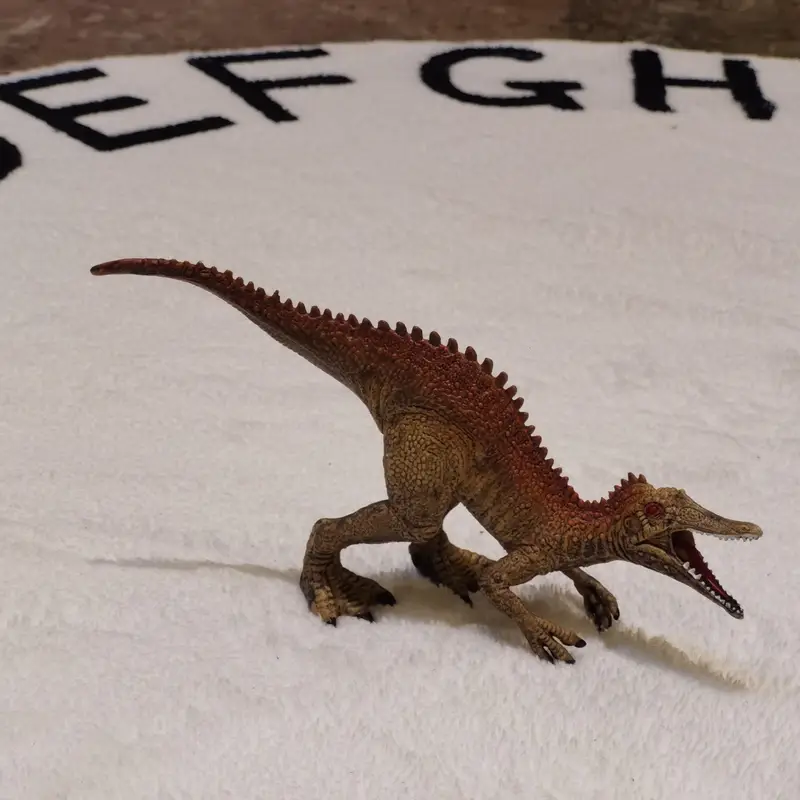The image depicts a plastic toy dinosaur standing on a white rug with big black letters "E," "F," "G," and "H" visible in the background, indicating it might be in a child's room. The dinosaur is depicted on its hind legs with small front arms, resembling a T-Rex. Its mouth is open, revealing a beak-like mouth filled with sharp teeth, and its head slightly resembles that of a pterosaur. The dinosaur features a detailed, scaly, and wrinkly brown texture with red spines running along its back and a long tail. The toy is leaning forward, as if crying out, with its tail raised in the air.